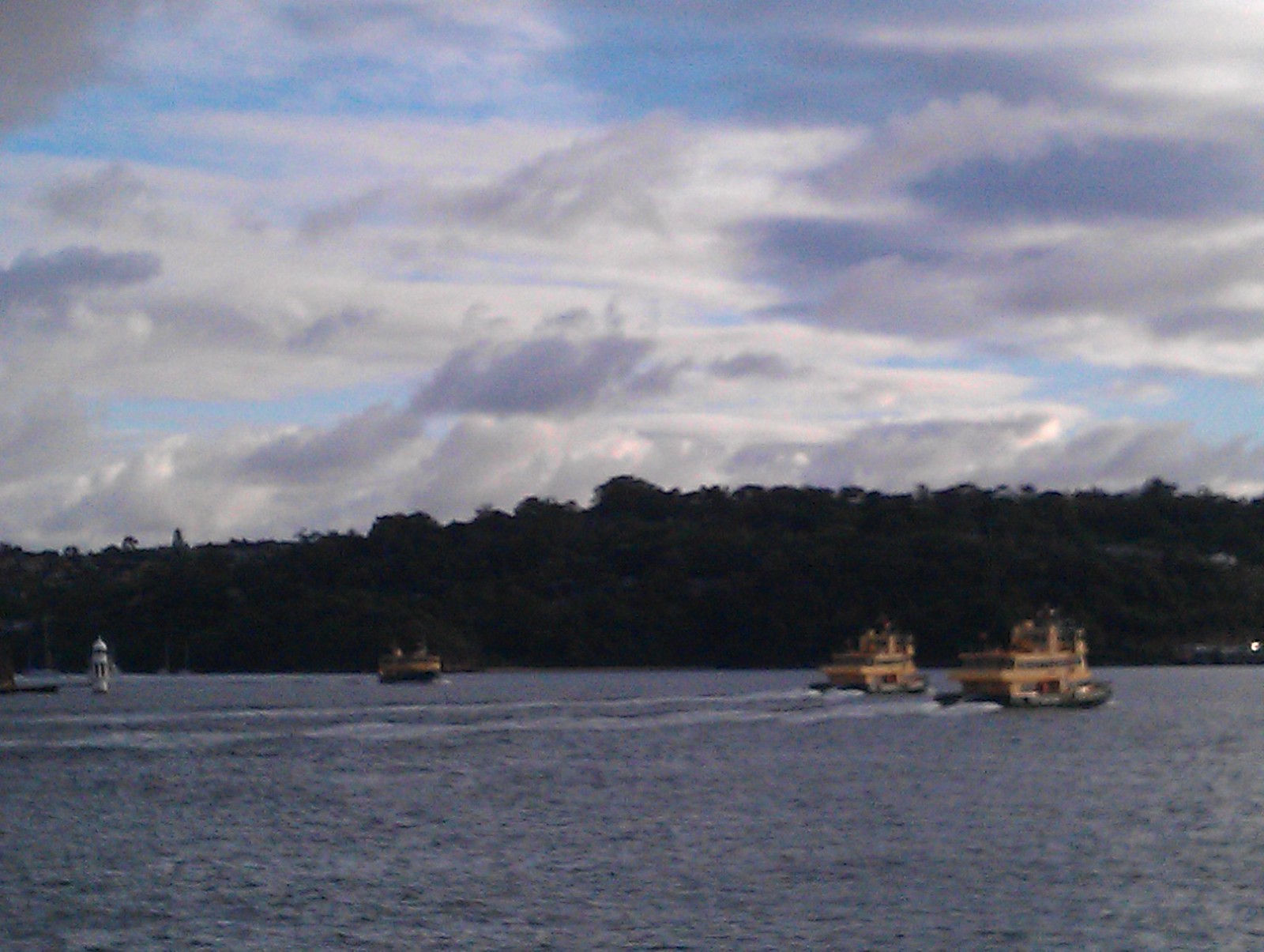The photograph showcases a serene daytime waterfront scene beneath a blue sky interspersed with large, wispy white clouds. Dominating the scene is a sizable body of lightly colored blue water, possibly an inlet of a lake, framed by a distant, ascending hillside blanketed in dense green forests. On the water are three boats, distinguished by their beige to orange hues with gray bottoms. Two of these boats are oriented northeast, while the third heads northwest. Adding a distinctive element to the scene is a small, tall, cylindrical white structure with a spire, situated in the left-hand portion of the image. Though its intended function remains unclear, it bears resemblance to a lighthouse. In the water, a white dinghy is also perceptible off to the left side. The photograph’s slight blur adds a touch of abstraction, enhancing the natural charm and tranquility of the waterscape amidst its natural surroundings.